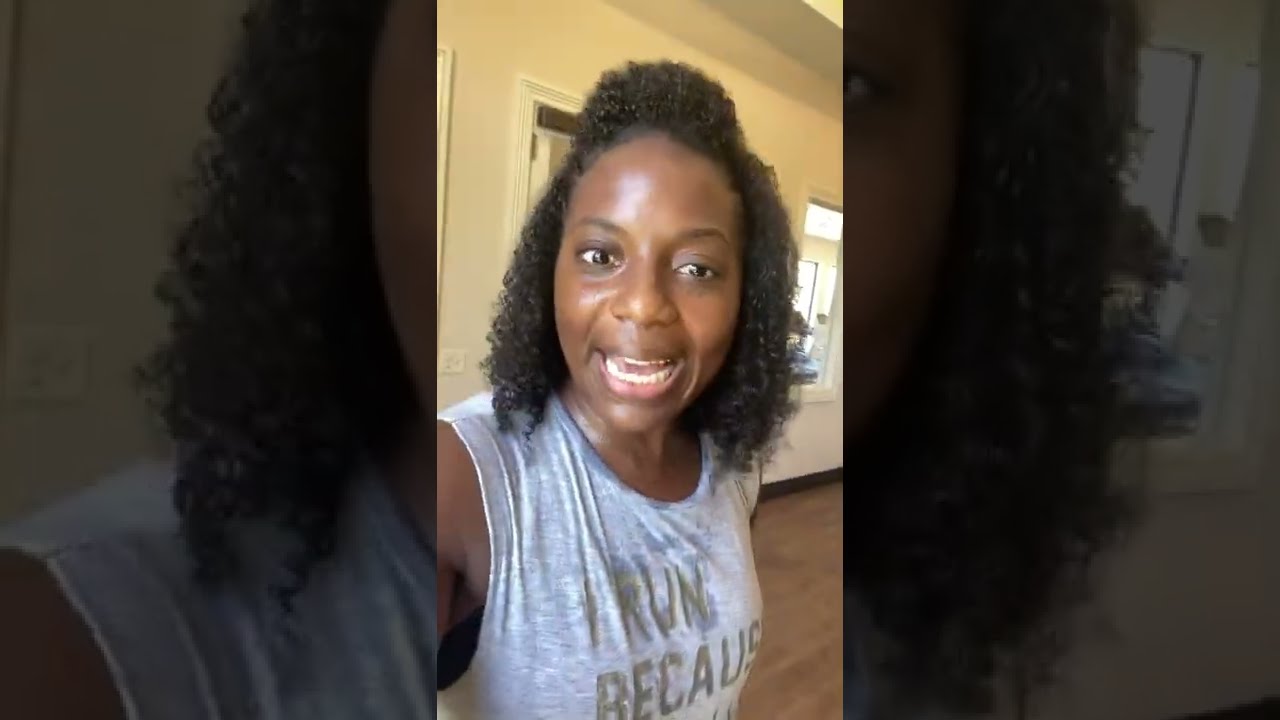A vibrant image captures a young African-American woman mid-speech, likely recording a video, possibly for a platform like TikTok. She has shoulder-length, kinky curly black hair that frames her expressive face. Her thin black eyebrows arch over bright eyes, and her mouth is open, revealing both rows of teeth, giving her a lively and earnest expression. She is clad in a sleeveless gray tank top, visibly damp with sweat, indicating recent physical activity. The shirt bears the partially visible slogan, "I run because..." and beneath it, she wears a black sports bra. Her skin, particularly around her neck and forehead, glistens with perspiration, further suggesting she has been exercising. The setting appears to be a clean, indoor space with dark brown wooden laminate flooring and a white wall equipped with doors and windows, probably indicating a room within a gym or a home. She is energetically detailing her recent workout, brimming with enthusiasm and high spirits.